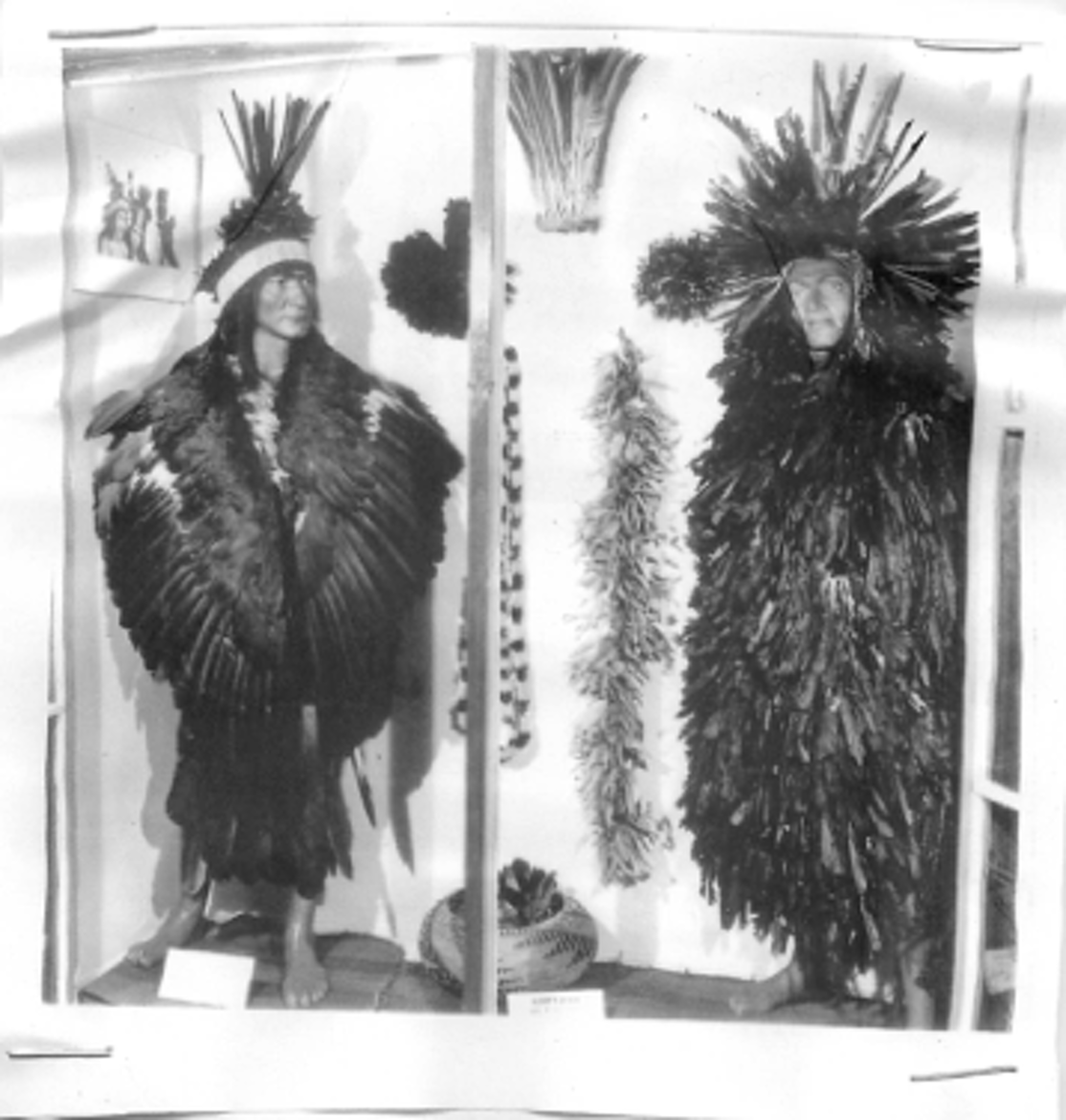This black-and-white photograph, slightly crumpled and possibly a printout, depicts two elaborately dressed Native American mannequins in what appears to be a museum display behind glass. The details of the photograph reveal a striking contrast between the two figures. On the left stands a female mannequin, posed facing forward with her head turned over her left shoulder, gazing to the right. She is adorned with an ornate feathered cape that resembles the wings of a bird, likely an eagle, with darker feathers underneath and lighter, grayish-white feathers above. Her attire includes a headband, from which a plume of feathers rises at the forehead. Her outfit is completed with a traditional Native American skirt that extends to her ankles, and she is barefoot.

On the right side of the photo is a male mannequin, standing slightly angled to the left but looking directly into the camera. His attire includes a heavily feathered garment that envelops him from shoulders to ankles, though unlike the female's garment, his lacks a distinct pattern, featuring a mix of dark and light feathers. He wears a headband crowned with an elaborate headdress featuring tall feathers that form a circular fan. Both mannequins are barefoot, enhancing the authenticity of their traditional dress. The photograph, though aged and showing signs of wear with wrinkles and staples at the edges, captures the intricate detail and artistry of Native American ceremonial attire, providing a captivating glimpse into cultural heritage.